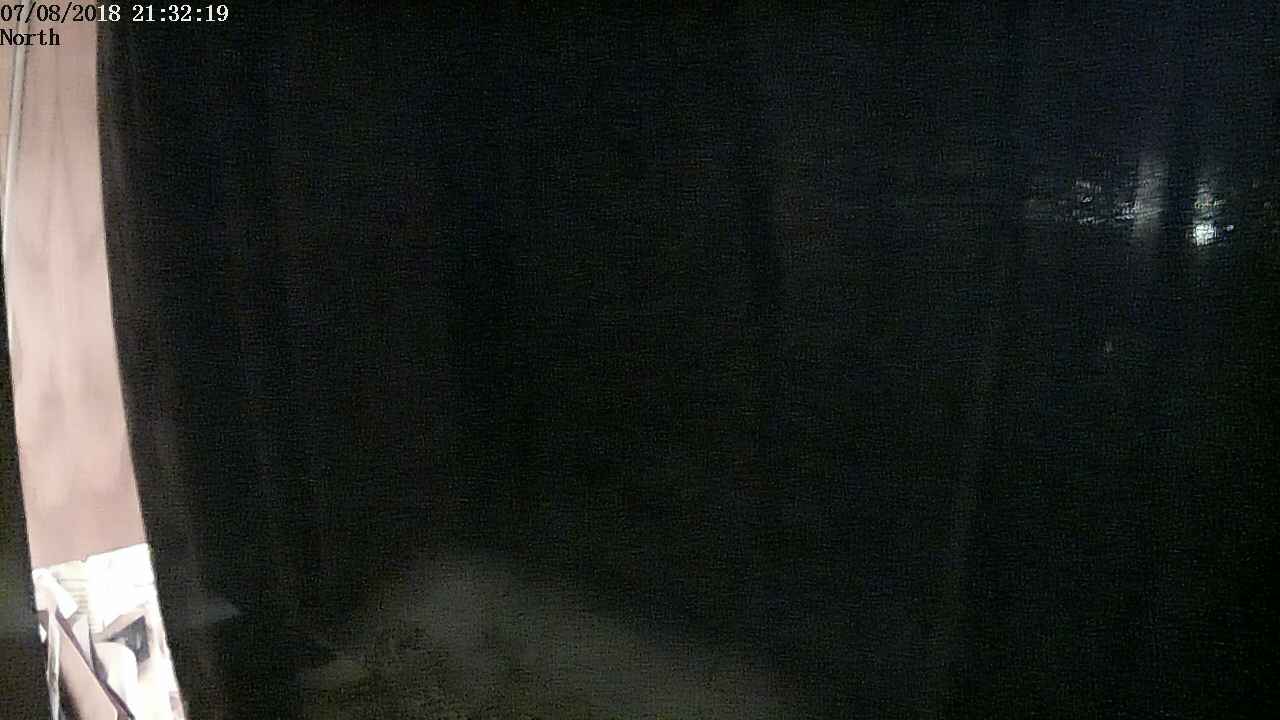A dark image captured by a security camera, dated 07-08-2018 with a timestamp of 21:32:19, is shown at the top of the frame. The word "North" is also displayed. The scene appears to be an outdoor area, possibly the entrance to a property, with the faint outline of a gating system and fencing visible. In the bottom corner, there's a brighter spot illuminating what seems to be a wooden pole, potentially with a small sign affixed to it. The overall image suggests the vicinity could be part of a residential building or home.